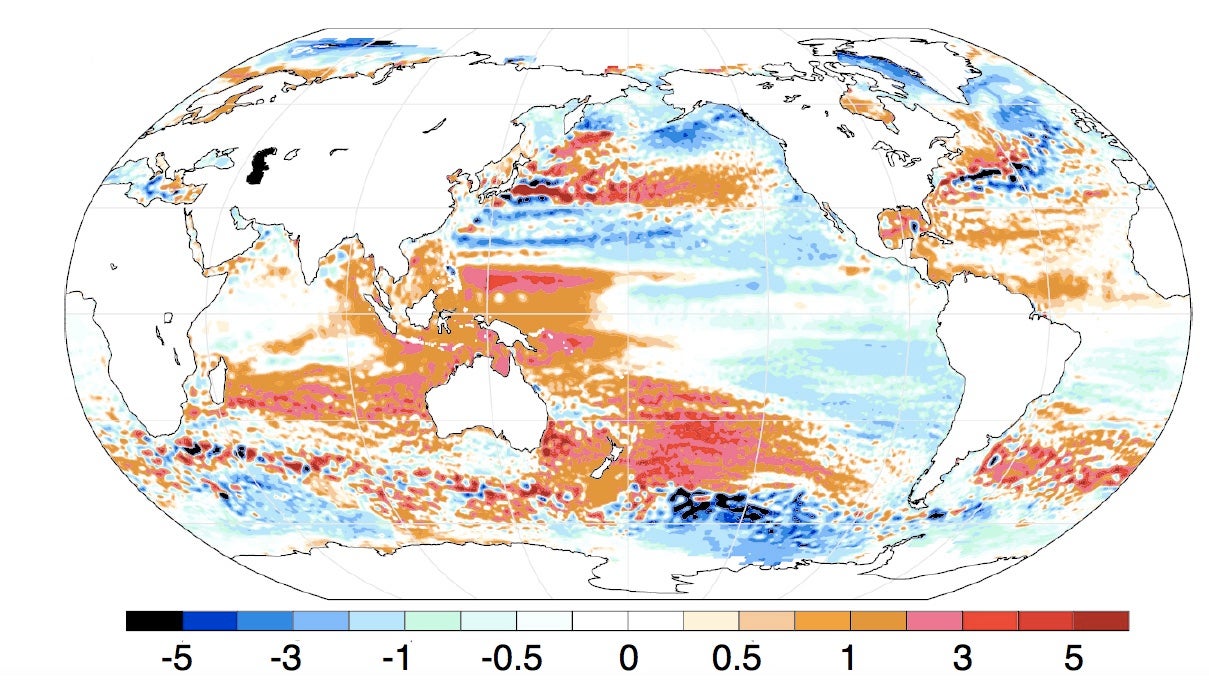The image is of a horizontally oriented, flat, oval-shaped map of the globe, showing various global data patterns in vibrant colors. The continents are depicted in black and white line drawings with distinct black outlines, while the oceans are filled with an array of hues including black, multiple shades of blue, mint green, cream, white, yellow, peach, orange, pink, red, and maroon. These colors correspond to a key or legend located at the bottom of the map, which indicates a numerical range from -5 to 5 with increments. This gradient key, marked by black text numbers, progresses from negative values in black and blue tones, through white at zero, to positive values in shades of red, depicting some form of metric – likely temperature changes or depths – across the geographic layout. The hot spots, particularly concentrated in the southern hemisphere, are highlighted in reddish-orange shades, suggesting significant data points in these regions. The map's detailed color coding facilitates a visual analysis of the specific global metric it is designed to represent.